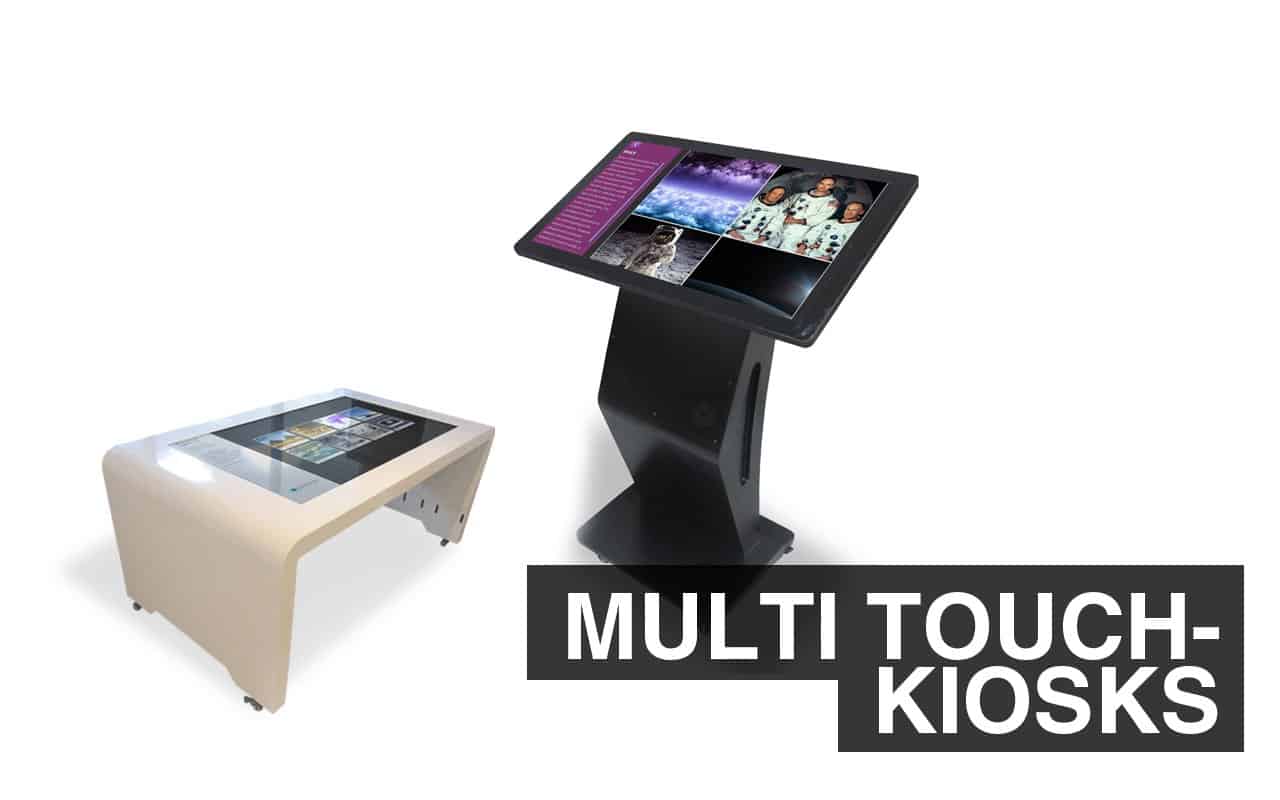The image is a detailed color illustration in landscape orientation, focusing on two distinct kiosks set against a white background, giving the appearance that they float. On the left, there is a short, three-sided rectangular table kiosk with curved corners, depicted in white. This kiosk appears to double as a bench and a table, featuring a monitor on top, angled towards the bottom left corner, and possibly equipped with castor wheels. 

In the center-right of the image stands a taller, podium-style kiosk with a black vertical base that extends in a triangular shape toward the bottom left. This black kiosk features a mid-waist height flat monitor with three distinct images displayed:
- Top right: An old photograph of astronauts in suits but without helmets.
- Bottom right: An area that looks completely black.
- Bottom left: An image of an astronaut on the moon, fully suited with a helmet, floating against a sky-like background with clouds.

Adjacent to this monitor, a purple section with white text is visible on the left side, although the text is too small to read clearly. At the bottom right corner of the image are the words "MULTI-TOUCH KIOSKS" in white capital letters inside two black horizontal rectangles. The overall style of the illustration emphasizes a 3D rendering with meticulous attention to typography and layout.